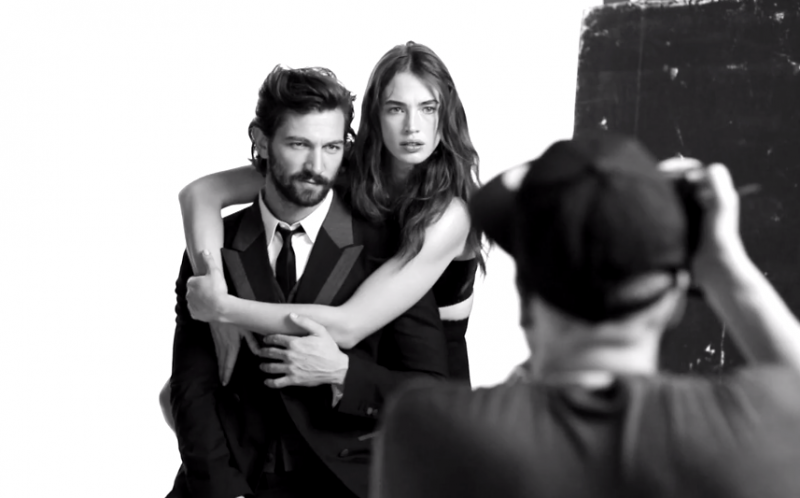In this black-and-white photo, a young man and a young woman are positioned intimately as part of a modeling shoot. The man, resembling a James Bond-like figure, is dressed in a tuxedo with a partially undone skinny black tie and a white shirt. He has dark brown hair and sits with a composed demeanor, his left hand gently resting on the woman's left forearm. The woman, who has long dark hair, is wearing a sleeveless black dress and stands close behind him, her arms wrapped affectionately around his shoulders. Both are looking towards the camera set up by the photographer.

In the foreground, the unfocused back of the photographer is visible. Clad in a baseball cap and a t-shirt, he holds the camera up to his face, fully engaged in capturing the scene. The background of the image is predominantly white, with an ambiguous dark structure on the right, possibly a trunk or a canister. This detailed and stylish composition emphasizes the classic and elegant atmosphere of the shoot.